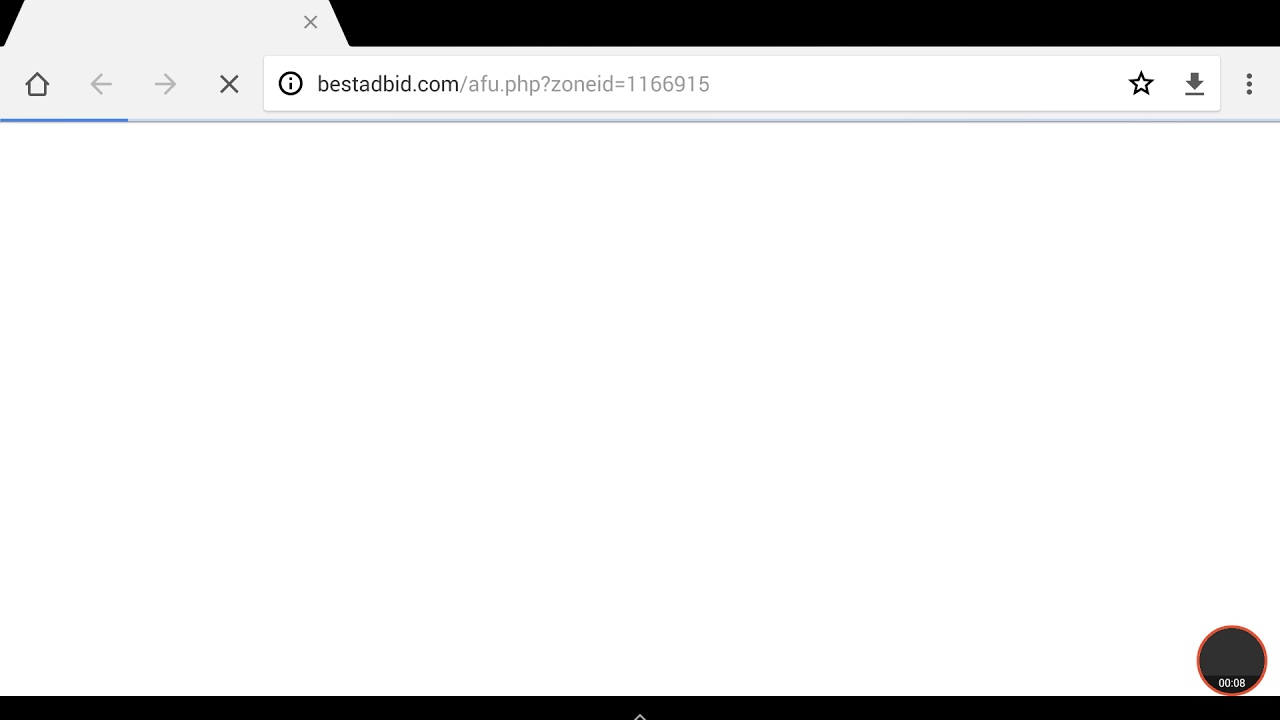The image is a screenshot of a web browser displaying a webpage. At the very top of the browser, there is a gray background featuring several navigation icons. On the left side, a home icon is visible, followed by a left arrow and a right arrow. To the right of these icons is a gray X.

Below this, in the URL bar, the web address is displayed as "bestadbid.com," with the additional query string "/afu.php?zoneid=1166915" shown in a lighter gray. On the right side of the URL bar, there is a gray star icon for bookmarking the page, a gray downward-pointing arrow for downloading, and a menu represented by three vertical dots.

Above the web address, the screenshot includes a black border without any visible content. Similarly, at the bottom of the browser, there is a black line. In the lower right corner, a gray circle outlined in orange contains the timestamp "00:08."